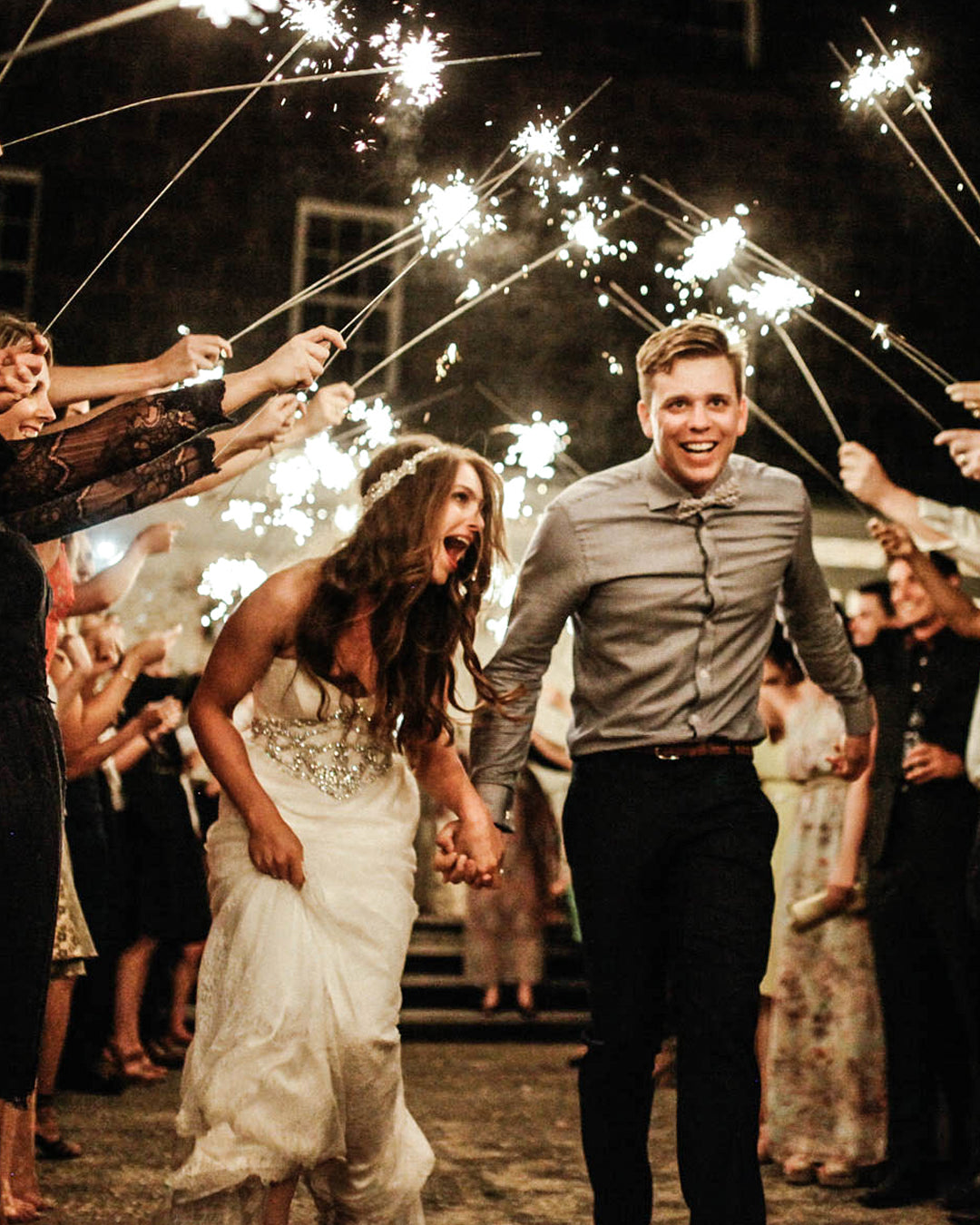This photograph captures an exhilarating moment as a newlywed couple exits their wedding ceremony. The bride, adorned in a white wedding gown and floral headband, her long brown hair cascading down her shoulders, beams with excitement. Beside her, her groom, dressed in a gray dress shirt and bow tie, with black pants, shares an ecstatic smile. They hold hands as they walk underneath a dazzling tunnel formed by their guests holding long, lit sparklers raised high to create a celebratory arch. Flanked by friends and family dressed in elegant attire, the couple is jubilantly making their first steps together into married life as they pass beneath the fiery canopy, set against a backdrop that includes a house and steps, symbolizing the start of their new journey.